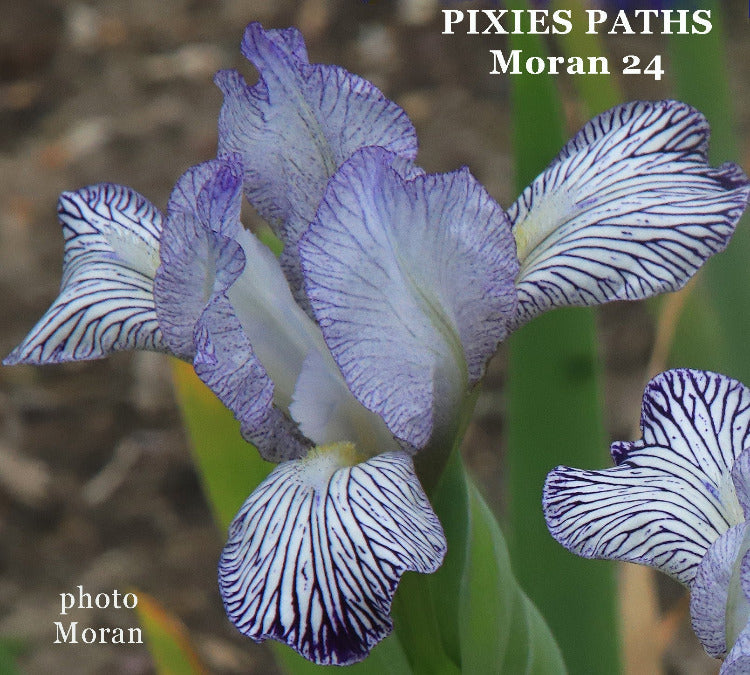This close-up photograph features a vibrant iris flower with a combination of violet-purple and white petals adorned with dark purple, vein-like lines. The center of the iris is a striking yellow with hints of white fuzziness. The flower's petals either droop downward or curve inward and outward, creating a dynamic structure. The leaves of the iris, in various shades of dark and light green, are visible but blurred, as is the brownish soil or leafy ground in the background. In the top right corner of the image, the text "Pixies Past, Moran 24" is visible in white, while "Photomoran" is inscribed in the bottom left-hand corner. The image captures the intricate beauty and delicate details of the iris, with the flower itself in sharp focus against the softly blurred surroundings.